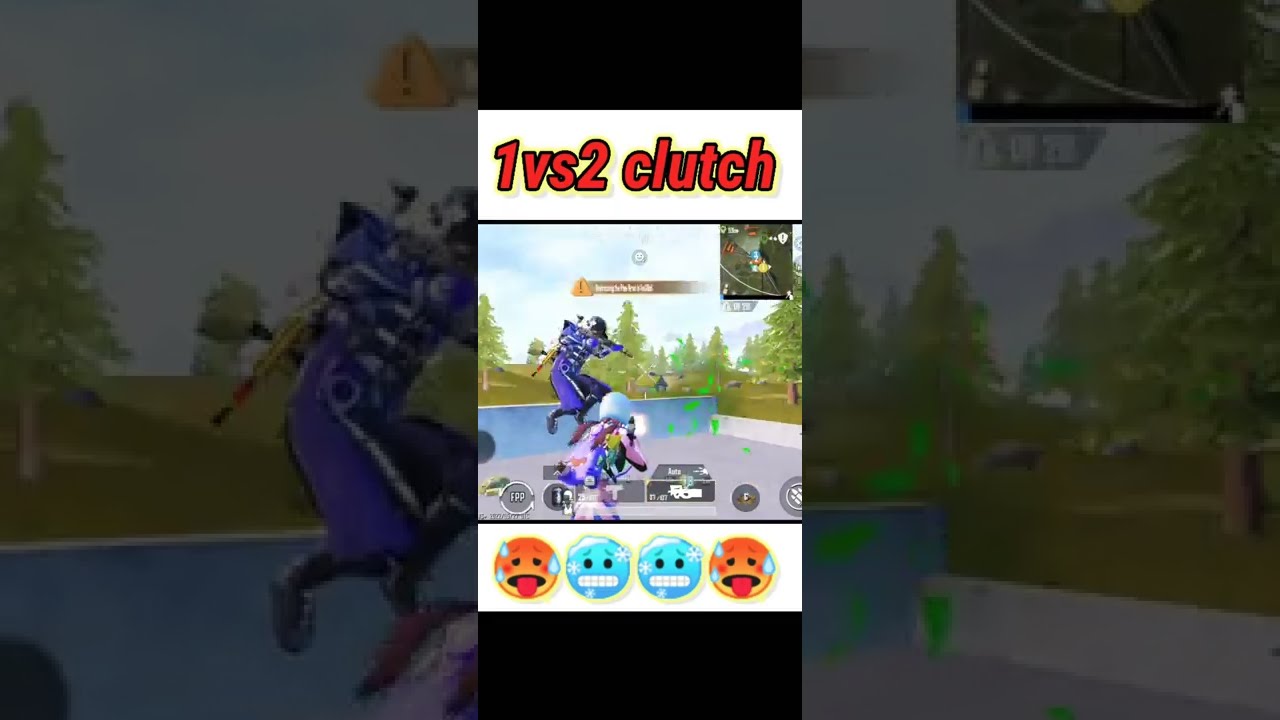The image is a video game screen grab in a landscape orientation with three panels. The left and right panels are grayed-out close-ups of the main middle image, which is in a vertical rectangle, likely from a mobile device. At the top of this central image, there is an orange banner with text that reads "One versus Two Clutch," indicating a gaming scenario. The image shows a 3D, third-person shooter scene, possibly from a game like Fortnite. Two characters are engaged in combat: the main character, a girl in a pink and black long-sleeve top with blue helmet and pigtails, and another character in blue armor and a black helmet. The girl is shooting at an opponent in front of her, with visible weapon flash. They appear to be on a rooftop, with cartoony forest and buildings in the background. At the bottom of the screen are four emoticon circles: the outer ones are orange, with their tongues sticking out and sweating, and the middle ones are blue, freezing with snowflakes. There's also a mini-map in the upper right corner of the screen and white bars with text at the top and bottom, contributing to the overall gaming interface.